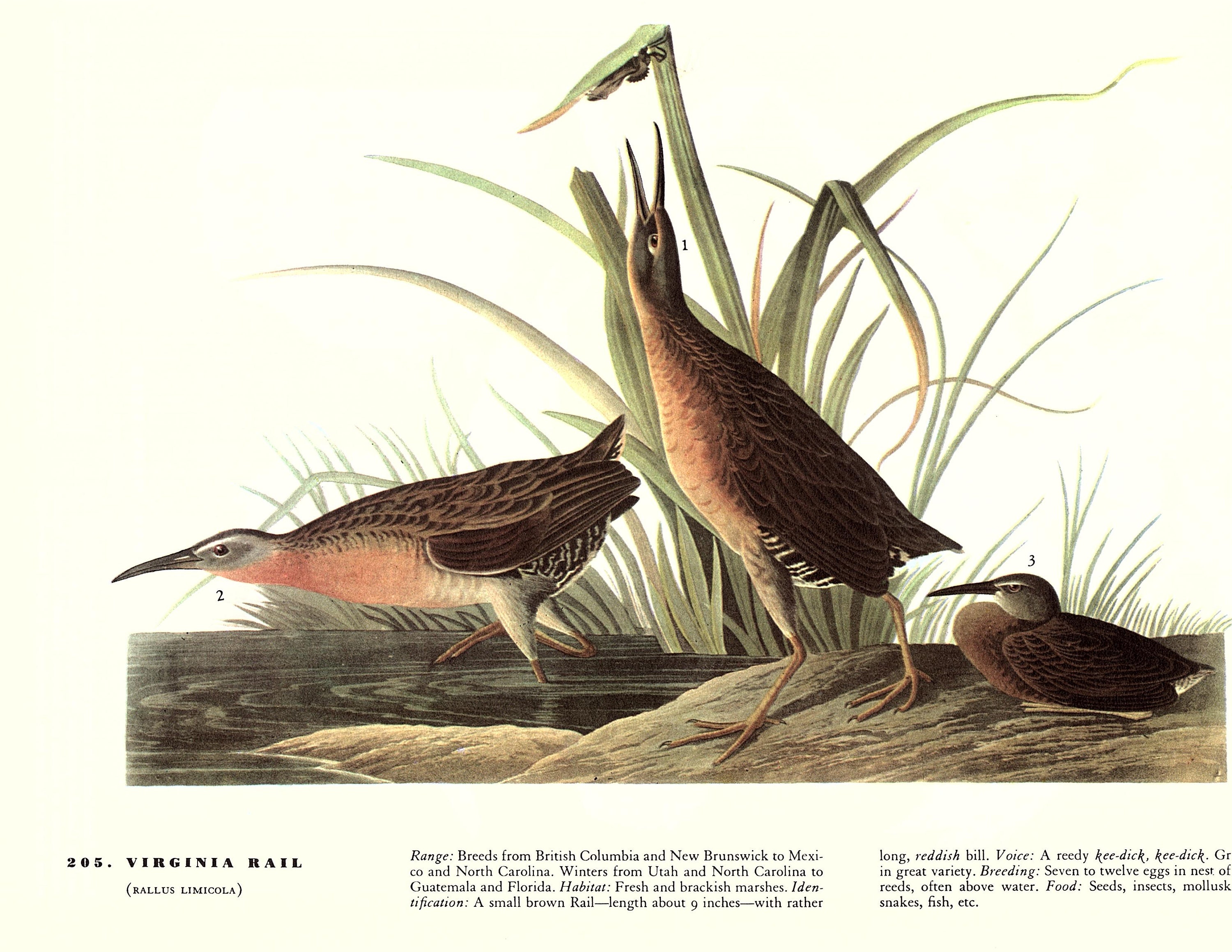This detailed artwork, labeled as number 205, illustrates the Virginia Rail, or Rallus limicola, and appears to be an informative page from a bird identification book or guide. The image, likely created using watercolor or acrylic paints, features three Virginia Rails in their natural habitat, standing at the edge of water with tall, green, reeded plants in the background. 

The bird on the left, identified as the male, is wading into the water, peering down as if searching for food. It has a long, pointed black beak, darker brown feathers, a rosy pink chest, and white legs. The central bird, depicted as the female, is standing on a small rock with its head stretched upward and mouth open, seemingly trying to catch an insect on the underside of a blade of grass. It shares similar features to the male but with slightly more brown coloring. The third bird, possibly a younger rail, is smaller, darker brown, and hunched down on the same rock, also facing left.

Below the image, detailed information about the Virginia Rail is provided, including its range, breeding from British Columbia and New Brunswick down to Mexico and North Carolina, and wintering from Utah and North Carolina to Guatemala and Florida. The text describes the bird's habitat, diet of seeds, insects, mollusks, snakes, fish, and more, making it a comprehensive representation of the Virginia Rail in both visual and textual form.